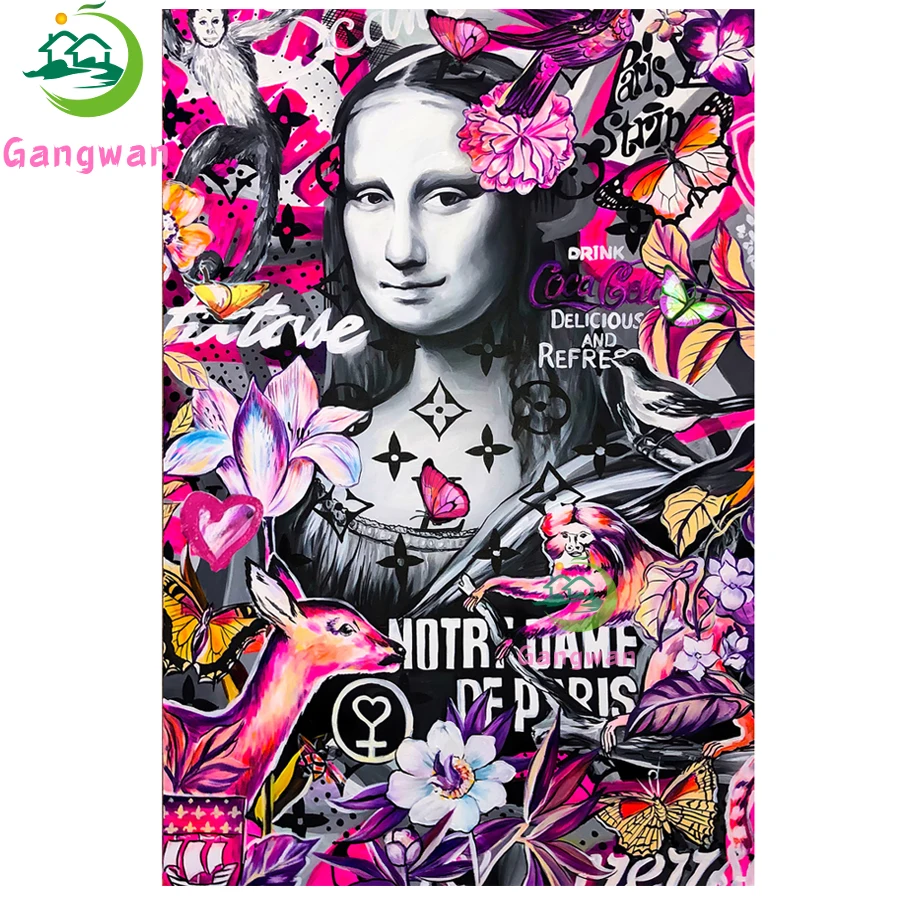The image is a detailed and vibrant collage painting with a horizontal rectangular format, resembling a cluttered poster. At the center of the composition, dominating approximately 50% of the space, is a black, white, and grey sketch of the Mona Lisa. She is surrounded by an array of colorful elements, primarily in pink, magenta, yellow, and orange hues. To her left, a baby deer painted in pink and magenta stands out, while above it, a grey and white monkey hangs from a stick. Various objects, such as butterflies, pink flowers, and pink hearts, are dispersed throughout the image, contributing to the vivid collage. Additionally, there is a Coca-Cola advertisement with the slogan "Drink Coca-Cola, delicious and refreshing." In the forefront, a green arc with a blue house inside, accompanied by the text "Gang War," adds another layer to the chaotic scene. Below the Mona Lisa, in white text, are the words "Notre Dame of Paris," hinting at a thematic connection to the renowned cathedral.